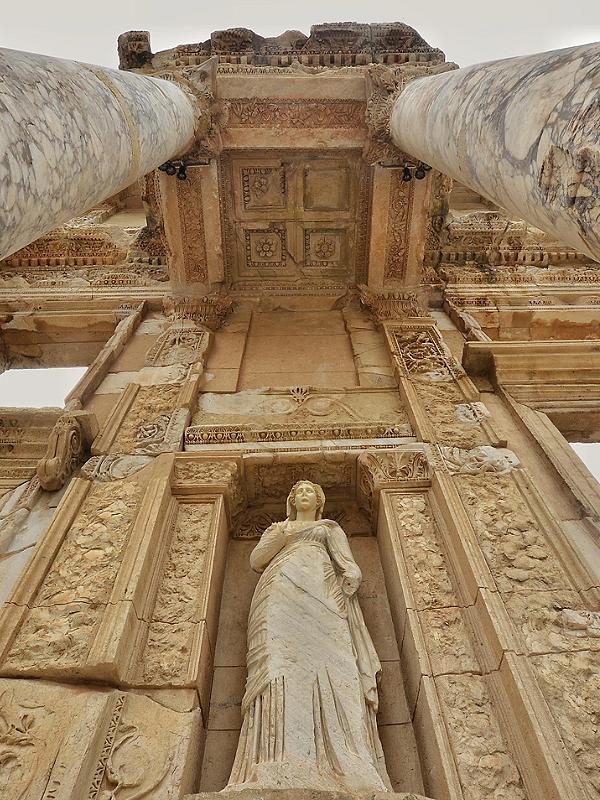The image captures a remarkable view of ancient ruins, resembling the iconic architecture of the Coliseum with its aged stone structures and weathered appearance. The perspective is strikingly unique, as the photo is taken from a low angle, seemingly from a position almost reclining beneath the remnants of an archway. In the composition, two large stone pillars rise majestically on either side of the frame, framing the scene. Above, the remains of an ornate stone slab wall are visible, complete with intricate carvings and patterns that have withstood the test of time. Between these pillars, centrally located, stands the statue of a woman clad in a flowing gown or robe, meticulously detailed despite the erosion that marks the surrounding stones. The backdrop includes the partially collapsed ceiling and hints of the sky, adding a sense of openness and antiquity to the scene. The stone surfaces, rendered in shades of tan and brown, are adorned with floral designs and elaborate carvings that speak to an ancient Roman artistic influence, portraying a sense of grandeur and historical depth.